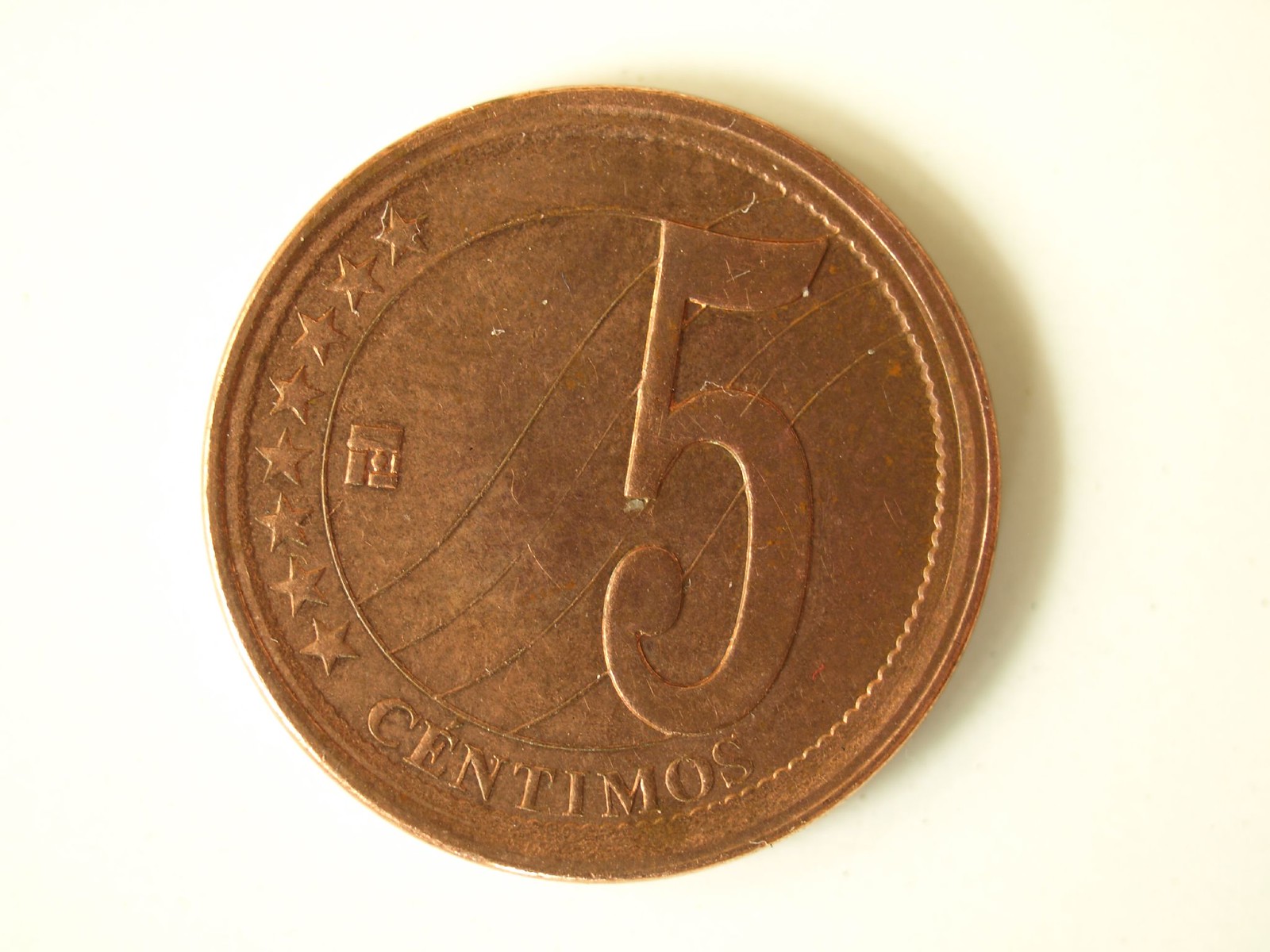This is a detailed close-up color photograph of an antique-looking coin with a rich copper or bronze patina, suggesting it has been in circulation for some time. Prominently featuring a large embossed number "5" which extends from the top to the bottom on the right-hand side, the coin also displays the embossed word "C E N T I M O S" at the bottom, indicating its denomination. On the left-hand side of the coin, there are eight five-pointed stars that are raised from the surface. Additionally, there is a small, square-shaped symbol towards the left. The center of the coin includes a thin circular design with three thin lines running across it. Although the coin's exact size is unclear, it appears to be roughly the diameter of a U.S. dime or penny.